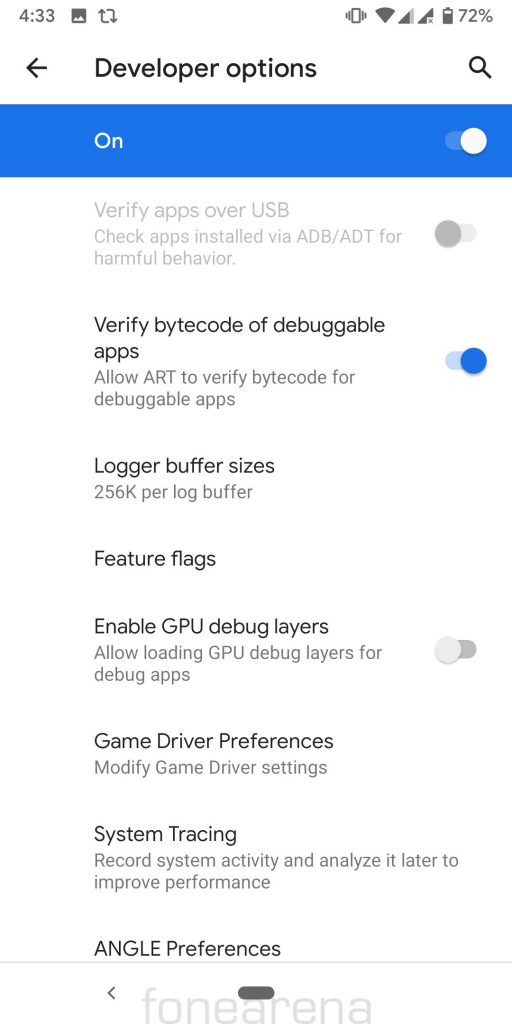This screenshot captures the "Developer Options" tab from a smartphone, displayed on a white background. At the top left corner, a black number "433" is visible beside a picture icon. An arrow stretches vertically up the left side and down across the bottom of the screen, then horizontally across the top, and down along the right side, where the battery level is shown at "72%." There is also a battery icon, followed by two internet connectivity icons, a Wi-Fi icon, and an icon indicating either an alarm or vibration mode.

Below the "433" on the left side, there is a bold black left-pointing arrow alongside text reading "Developer Options." On the top right, there is a black search icon (magnifying glass). A blue border runs straight down from the "D" in "Developer," with the word "On" in white text, indicating the toggle is enabled. Underneath this, in light gray, three lines are visible indicating a toggled-off setting, followed by another toggled-on setting confirmed by "TE code of debuggable apps."

Further down, several settings are listed:
- A black text option reads "Allow ART to verify bytecode for debuggable apps," which is toggled on with a blue switch.
- "Logger buffer size" in black text, accompanied by descriptive information.
- "Feature flags" section.
- "Enable GPU debug layers," indicated by a toggled-off switch.
- "Game driver preferences," followed by a line underneath.
- "Systems tracing" with descriptive information.
- "ANGLE preferences," which extends beyond the visible portion of the screen.

The bottom of the screen is slightly faded with the text "Phone Arena" depicted in black.